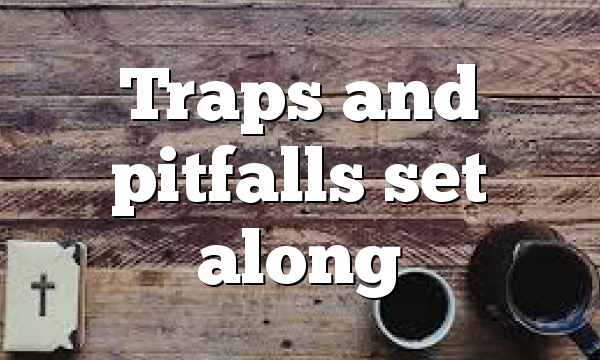The image is an overhead shot of a worn, weathered wooden table, possibly a picnic table, marked with scuffs, displaying various shades from light tan to dark brown, and sprinkled with spots that appear to be dirt or damage. Prominently displayed across the center of the image in bold, white capital letters are the words "Traps and pitfalls set along." In the bottom left corner, there is a small, tattered Bible with a gray cover and a dark cross on its front. On the bottom right, an old-fashioned dark blue pitcher mug sits next to a white coffee cup, filled nearly to the brim with a black substance presumed to be coffee. This graphic art piece emphasizes the contrast between the rustic, damaged wood and the stark, bold lettering.